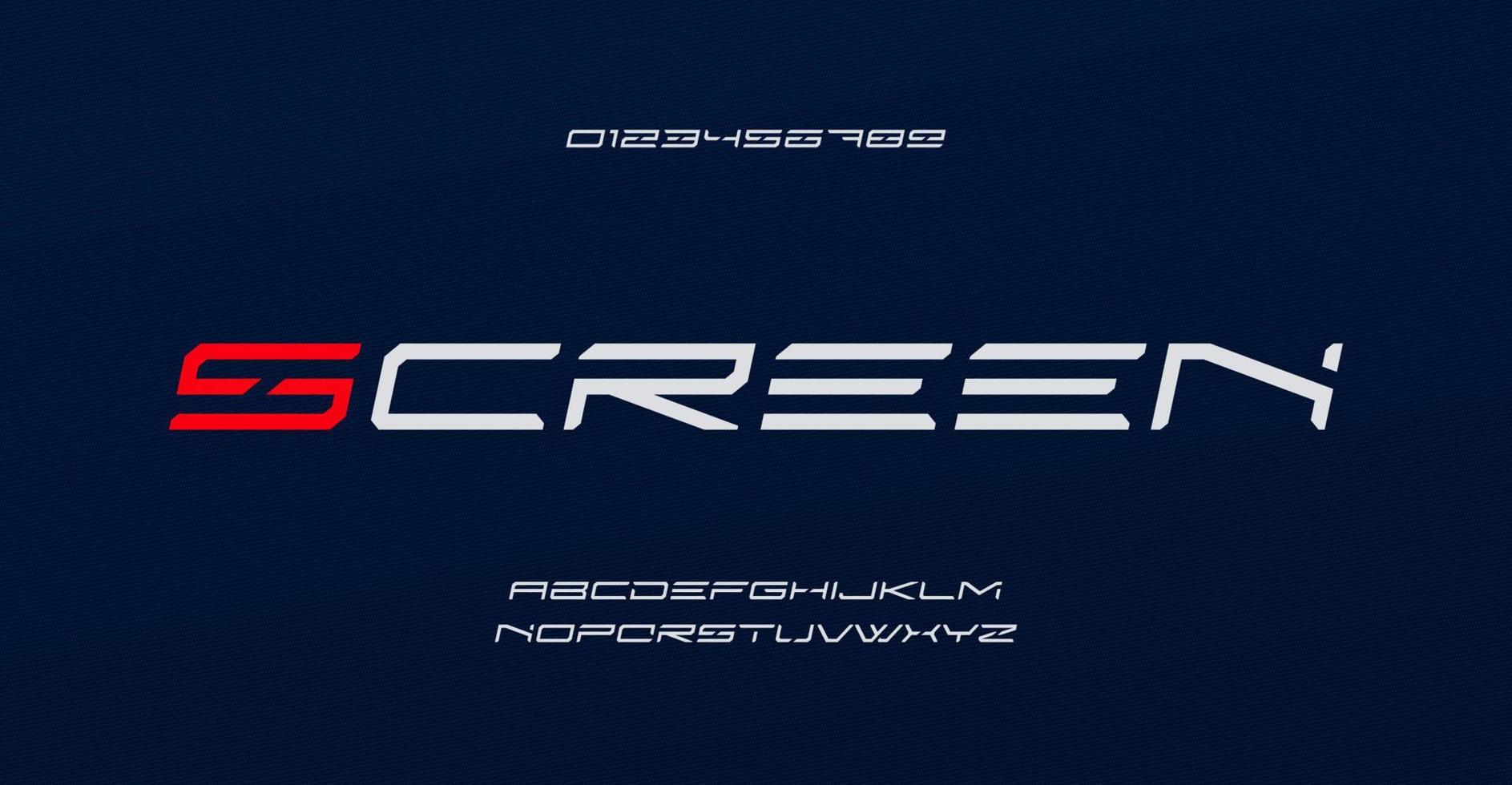The image appears to be a demonstrative screenshot or an advertisement showcasing a unique font. The background is a dark navy blue, and the content is centrally aligned. At the top, in a single line, the numbers "0 1 2 3 4 5 6 7 8 9" are displayed in this specific font. Below, the word "SCREEN" is prominently featured with a red "S" and the remaining letters in white. The font is characterized by some missing lines at the ends of the letters, giving it a distinctive, obtrusively artistic appearance. Beneath the word "SCREEN" is the entire alphabet "A-Z" displayed in the same font, maintaining the same style. The font's peculiar design and alignment indicate that this image serves as a demonstration or an advertisement for this particular font type.